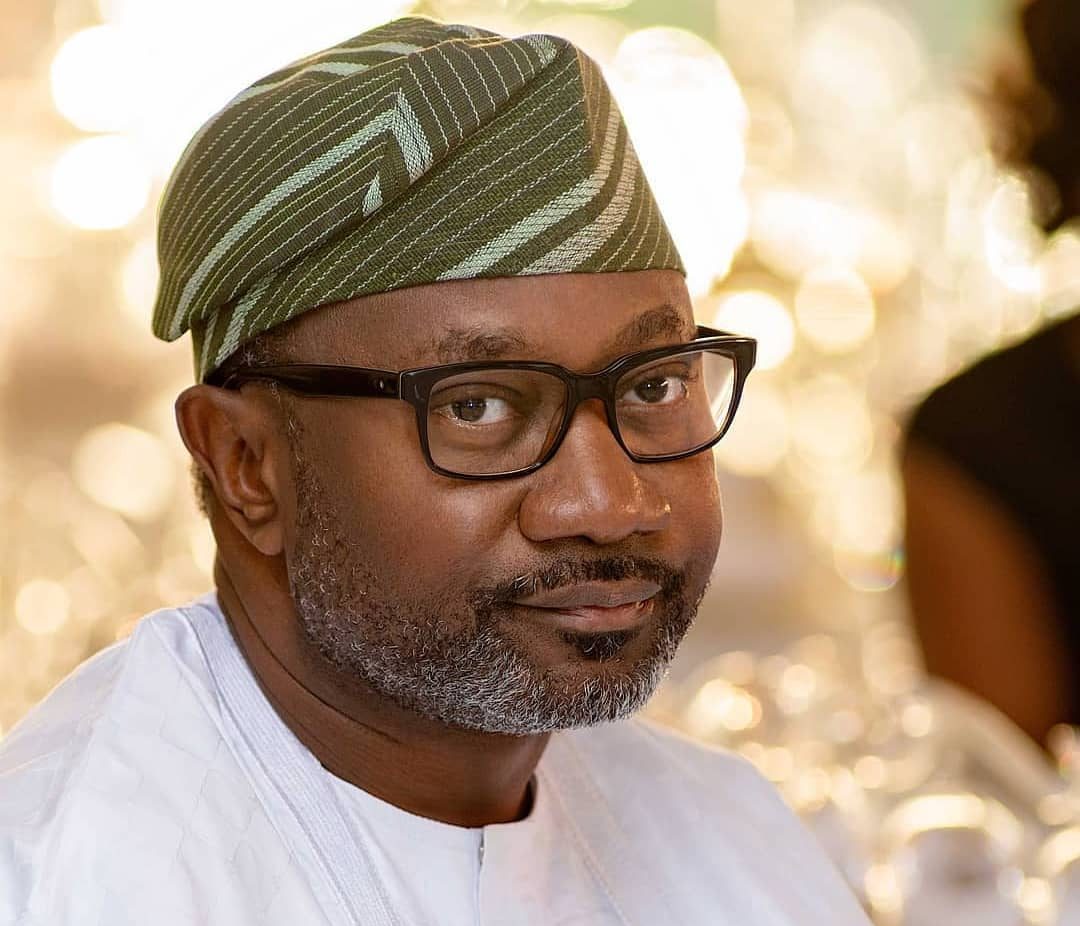The image depicts an African-American man, seemingly in his early 40s, with a mustache and a salt-and-pepper stubble. He is wearing modern black-rimmed glasses and has brown eyes. His attire includes a white shirt, and on his head, he dons a woven cap with olive green and white stripes, possibly indicative of his religious or cultural background. The man is looking towards the camera with a composed, perhaps slightly amused expression. In terms of view, we see him from his shoulders up, revealing his right ear. The background is a soft, out-of-focus gold, with indistinct lighter areas and blurred elements, including part of another person’s arm and head, which also appear to be African-American. The overall atmosphere focuses warmly on the man's serene visage against the indistinct, but warmly lit, backdrop.